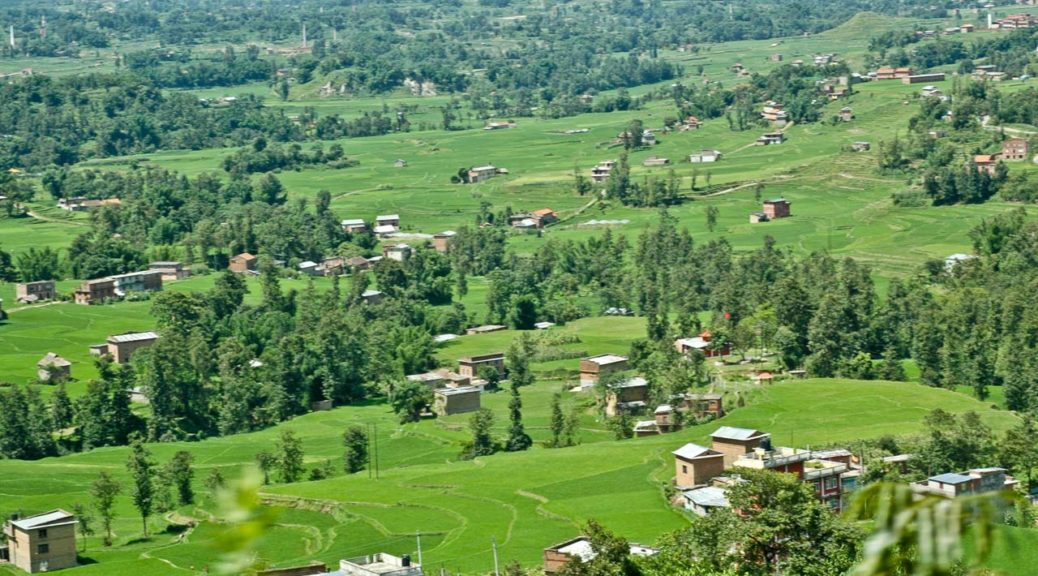This horizontal, rectangular photograph captures a lush, verdant countryside landscape viewed from a high vantage point, possibly from a hill or an airplane. The image showcases a picturesque valley setting abundant with vibrant green fields and dotted with small, squarish houses predominantly light tan or brownish in color, featuring white roofs. The landscape gradually increases in elevation towards the top of the image, suggesting a transition into hilly or mountainous terrain. Bountiful tall green trees line the scene, especially clustering around the houses, creating a harmonious blend of nature and habitation. There are approximately 50 houses scattered throughout the image, some nestled closely together in clusters, particularly noticeable in the lower right and central areas of the photograph. Roadways are scarcely visible, partially hidden by the dense foliage, emphasizing the lush, uninterrupted green expanse. The daylight illuminates the scene brightly, indicating a sunny, warm day.